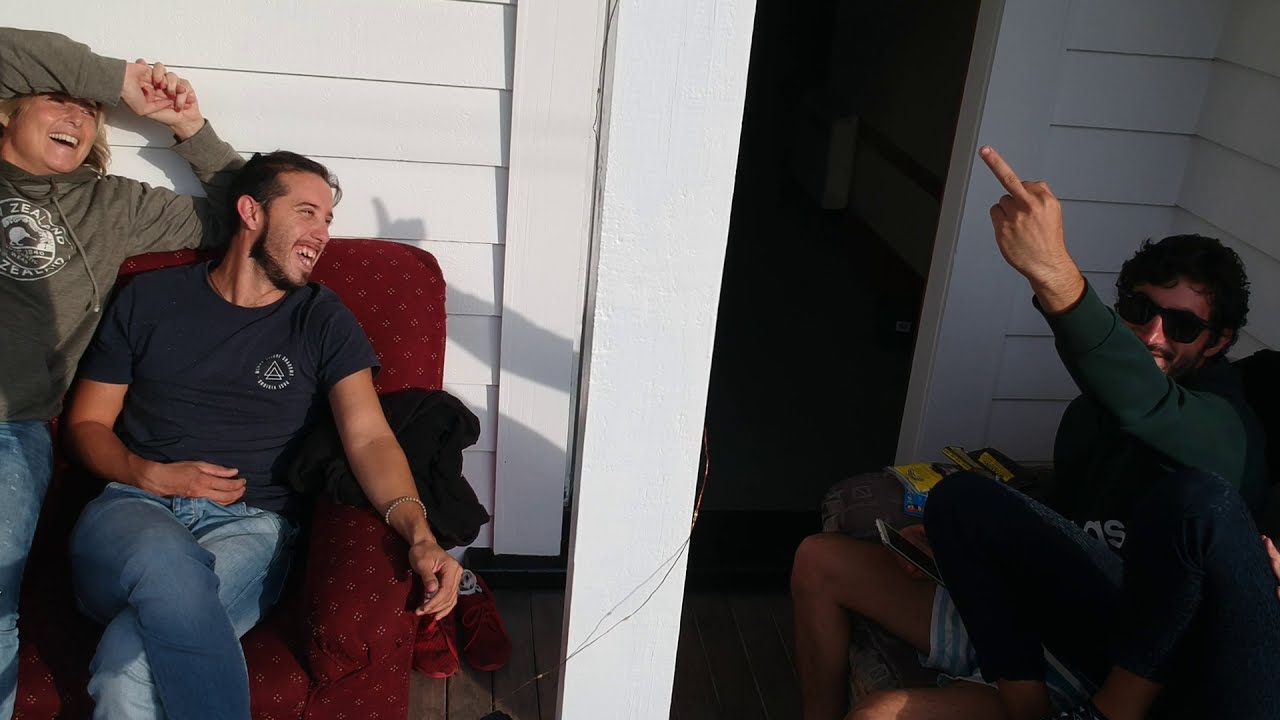In this photograph, three people are relaxing on a wooden porch of a house with white, horizontal wood-paneling. The scene is bathed in the warm, slanted light of the late afternoon sun, suggesting it is near sunset. Central to the image is a white, painted column, and behind it, a doorway leading into the dark interior of the house.

On the left, a blonde woman dressed in a gray sweatshirt and blue jeans sits on a red couch. Next to her, a man with long dark hair and a beard, wearing a navy t-shirt and blue jeans, is seated. Both are laughing heartily. Opposite them, to the right of the image, is another man lounging on a gray sofa chair. He sports a green sweatshirt, white and light-blue striped basketball shorts, and dark, horn-rimmed sunglasses. He completes the scene with a mischievous expression, flipping off the camera with his middle finger.